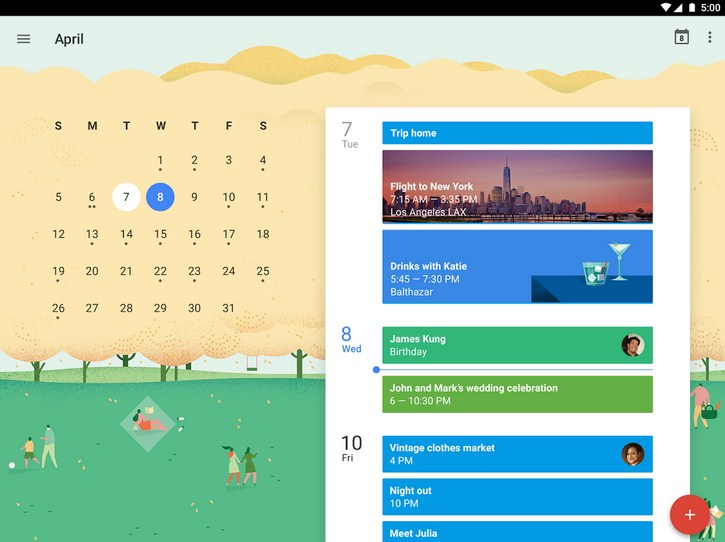A person is looking at their Google Calendar on a desktop display. In the upper left corner, three black lines indicate a drop-down menu. To the right, "April" is displayed in bold black lettering. Surrounding the calendar is a clip art cartoon scene of a park. The top portion features a large beige and yellow area representing tree leaves, with green tree trunks extending downward. At the bottom, there is grass and various people laying down, playing soccer, and walking together.

In the orange area, symbolizing tree tops, bold black initials "SMTWTFS" mark the days of the week. The calendar grid begins with a black "1" under Wednesday (W) and continues up to "31" under Friday (F). The number "6" is marked with two dots beneath it, while "7" is highlighted with a white circular background. The number "8" is also distinct, featuring a dark blue background and white text.

On the right-hand side, there is an overlay with a white rectangular area. At the top of this overlay, a blue strip with white text reads "Trip Home." Below it, a banner displays a cityscape during sunset with "Flight to New York" written in white on the left. Beneath this, the text "7:15 AM - 3:35 PM Los Angeles LAX" is shown in capital letters.

Further down, another section with a blue background and a dark blue table includes a cartoon image featuring a wine glass and a cup on the right. In bold white text, it says "Drinks with Katie," followed by "5:45 - 7:30 PM" in non-bold text. The final line reads "Balthazar" (with proper capitalization).